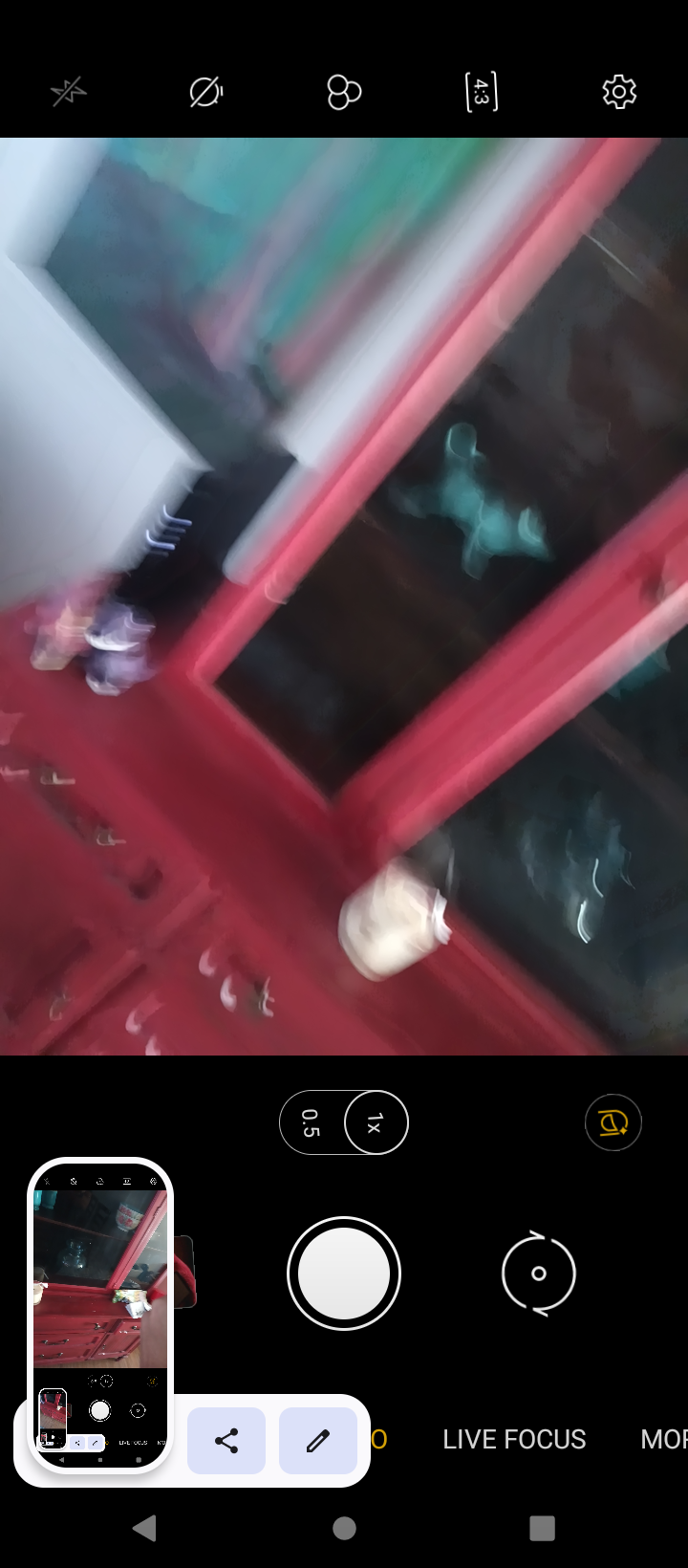The image depicts a blurry photo taken with a smartphone in portrait mode, focusing on a red wooden cabinet with glass doors, containing various household items. Displayed prominently in the bottom left corner is a clearer, previously taken screenshot of the same scene. The composition suggests a person photographing their phone screen, capturing both the phone's top black status bar and bottom control pad. The cabinet's contents include coffee mugs, glass bowls, and a porcelain dog, while the scene is set against a white wall with a slightly skewed perspective. This unique setup offers a juxtaposition of a blurred live view and a clear screenshot, emphasizing the red cabinet's design with its gold handles and glass doors.